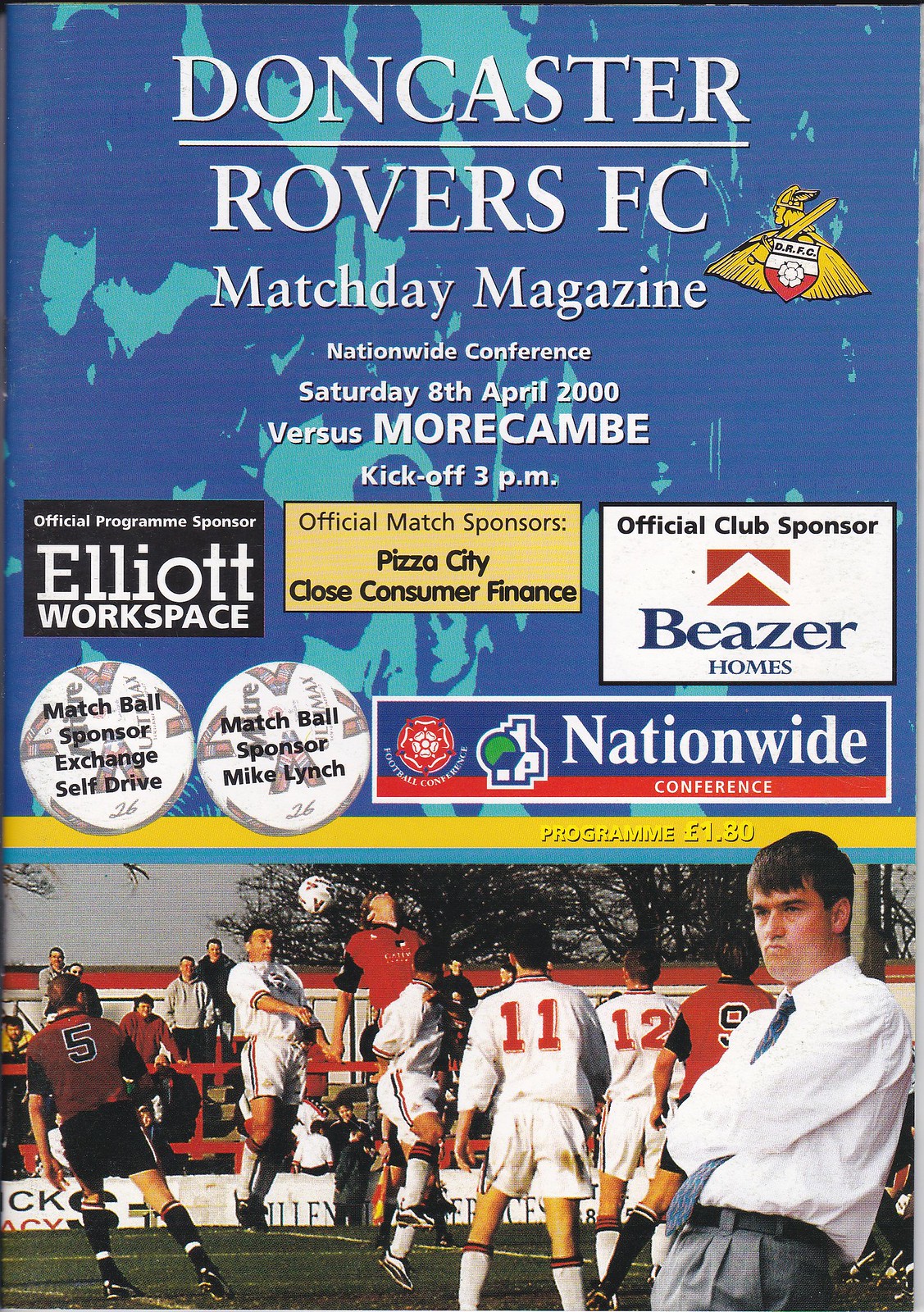The magazine cover features a vibrant and detailed layout that captures the essence of a pivotal football match. The top portion of the cover is adorned with a dark blue background interspersed with lighter blue shapes, and in bold, white uppercase text, it prominently displays "DONCASTER ROVERS FC," with an underlined title. Adjacent to this, on the right, there is a logo of the team, depicting a helmet with wings holding a sword over its shoulder.

Below the main title, a series of details unfold in white uppercase letters: "MATCHDAY MAGAZINE" followed by "NATIONWIDE CONFERENCE," the date "Saturday, 8th April 2000," and the match-up "VERSUS MORECAMBE," with the kickoff time "3 P.M." Following this, a structured grid of sponsors is presented. 

The first sponsor box on the left, marked as the "Official Programme Sponsor," features "ELLIOTT WORKSPACE" in white text on a black background. The center box highlights the "Official Match Sponsors," listing "PIZZA CITY" and "CLOSE CONSUMER FINANCE" in yellow. The right box identifies the "Official Club Sponsor," displaying a logo and the name "BEEZER HOMES."

Further down, a blue banner with two logos runs horizontally, denoting the "Nationwide Conference." Set against this backdrop are two white soccer balls indicating the "Matchball Sponsor" roles: the first ball names "EXCHANGE SELF-DRIVE," and the second names "MIKE LYNCH."

At the bottom of the cover, a dynamic photograph captures live action from the football field, featuring players in white and red uniforms actively engaged in a match. Overlaid on this scene, a man dressed in a long-sleeved white shirt and a tie, likely the manager, leans pensively against a surface, adding a human element to the energetic background of the game.

In the lower section of the design, the magazine's details wrap up with a white banner across the entire width, indicating the price as "Programme £1.80." This comprehensive cover encapsulates the anticipated face-off in the Nationwide Conference, emphasizing the event and its sponsors with striking visual and textual elements.